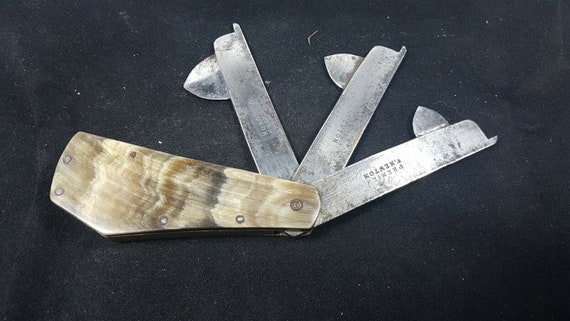This landscape-oriented photo features a black, grainy background with various white spots and a few thin gray hairs scattered across the surface. At the center of the image is a unique Swiss Army knife. The knife's handle is crafted from wood, showcasing a streaky grain pattern in shades of dark brown, light brown, light gray, and a hint of yellow, interspersed with some black and gray tones. The handle is affixed with five screws—four smaller studs and one larger screw.

Prominently extending from the wooden base are three equally spaced metallic blades. Each blade is a long rectangle with a sharp, pointed tip. Additionally, each blade features a wider, arrowhead-like protrusion on the side, with these arrowheads varying in size from small to larger, creating a layered effect. The intricate design also includes some metal hardware embedded in the handle, adding to the functional aesthetics of the knife. The surface beneath the knife appears to be a cloth material, contributing to the textured depth of the overall composition.